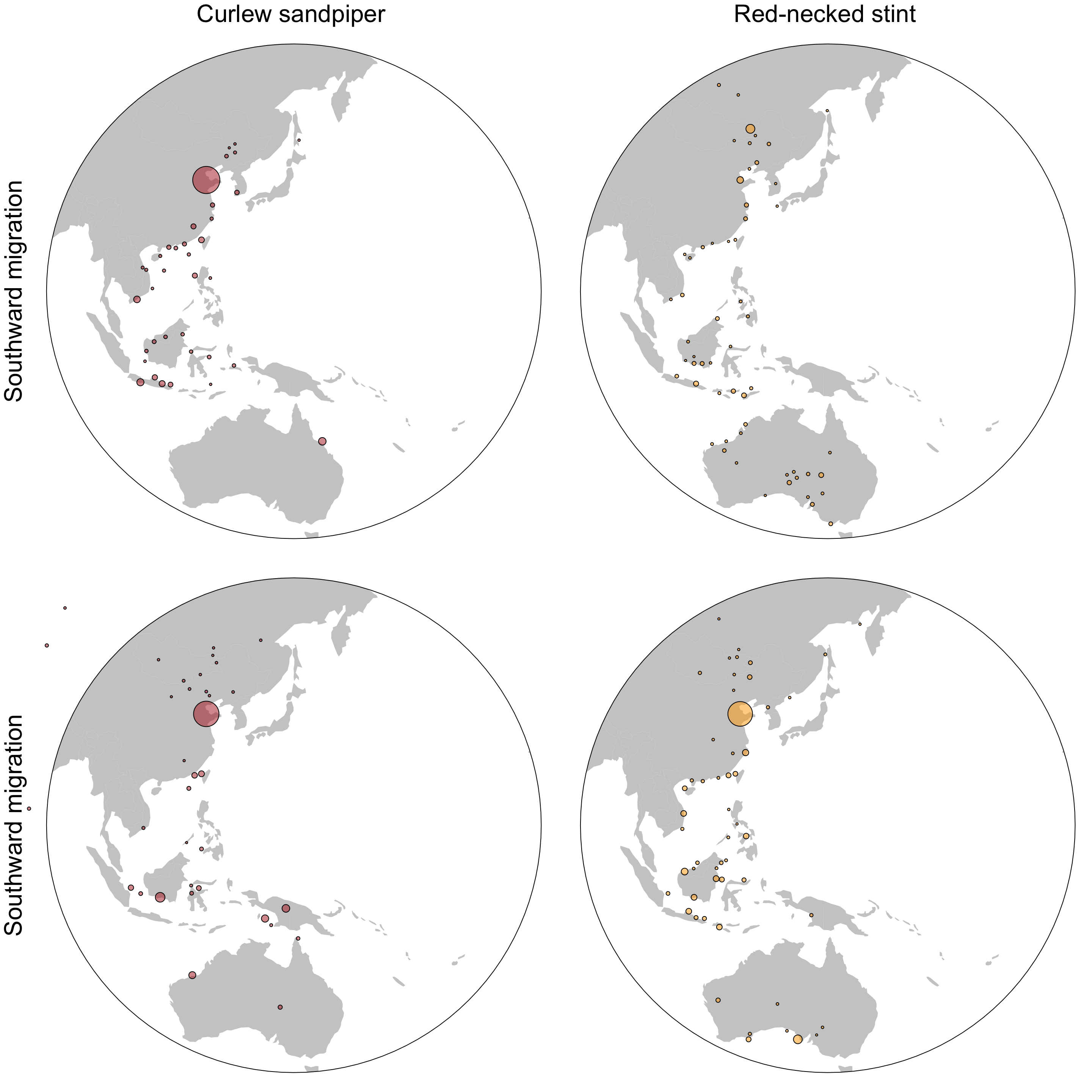The image is a detailed, black-and-white technical illustration composed of four globes arranged in a grid, representing the southward migration patterns of two bird species: the Curlew Sandpiper and the Red-necked Stint. Each quadrant in the grid features a simplified circle depicting part of the Earth's surface, focusing on the region encompassing Eastern Asia, Southeast Asia, and Australia. 

The left column is labeled "Curlew Sandpiper" and includes two globes showing this species' migration patterns with red dots. One map illustrates large concentrations near India, China, and Japan, as well as smaller clusters throughout the South Pacific islands and Australia. The right column, titled "Red-necked Stint," displays smaller yellow dots indicating this species' migration routes. Each species' row displays southward migration patterns, yet the specific dot placements vary between the rows, signifying different migratory stops for each species within the same region.